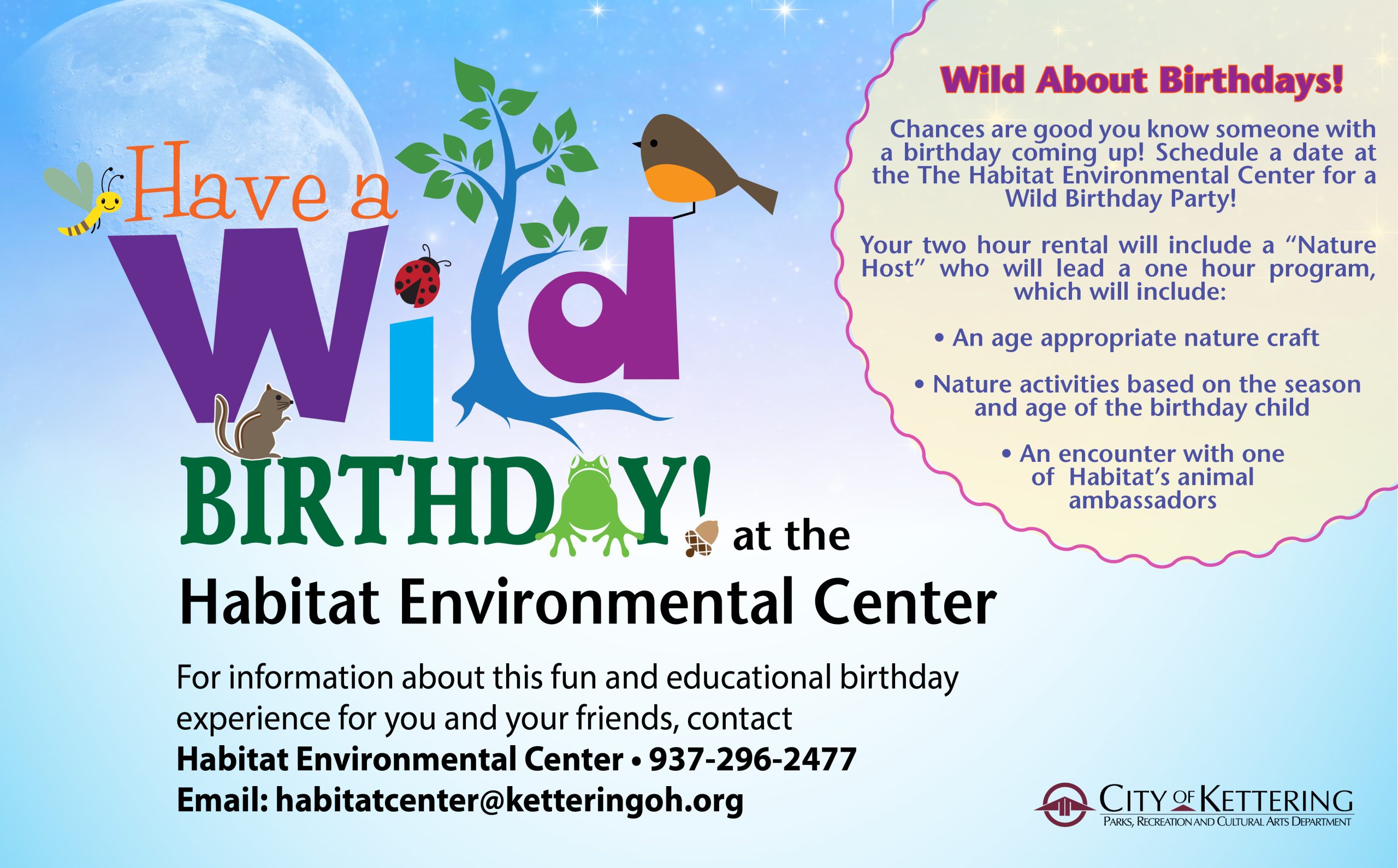This detailed banner advertises a wild birthday party experience at the Habitat Environmental Center, City of Kettering. The sky-blue background features a powder blue sky with a moon silhouette in the upper left corner. Prominent at the top, the text reads "Have a Wild Birthday at the Habitat Environmental Center," with the word "wild" creatively designed: a yellow bug with wings forms the letter "H", "W" is in purple, "I" in blue with a ladybug as the dot, "L" shaped as a blue tree with leaves, and "D" in purple with a bird perched on it. 

A detailed description follows: "Chances are good you know someone with a birthday coming up. Schedule a date at the Habitat Environmental Center for a wild birthday party." The poster highlights the features of the two-hour rental including: a nature host leading a one-hour program, age-appropriate nature crafts, seasonal nature activities, and an encounter with one of Habitat's animal ambassadors.

For more information or to schedule, it advises contacting the Habitat Environmental Center at 937-296-2477 or emailing habitatcenter@ketteringoh.org. At the bottom right, it proudly displays the City of Kettering logo.